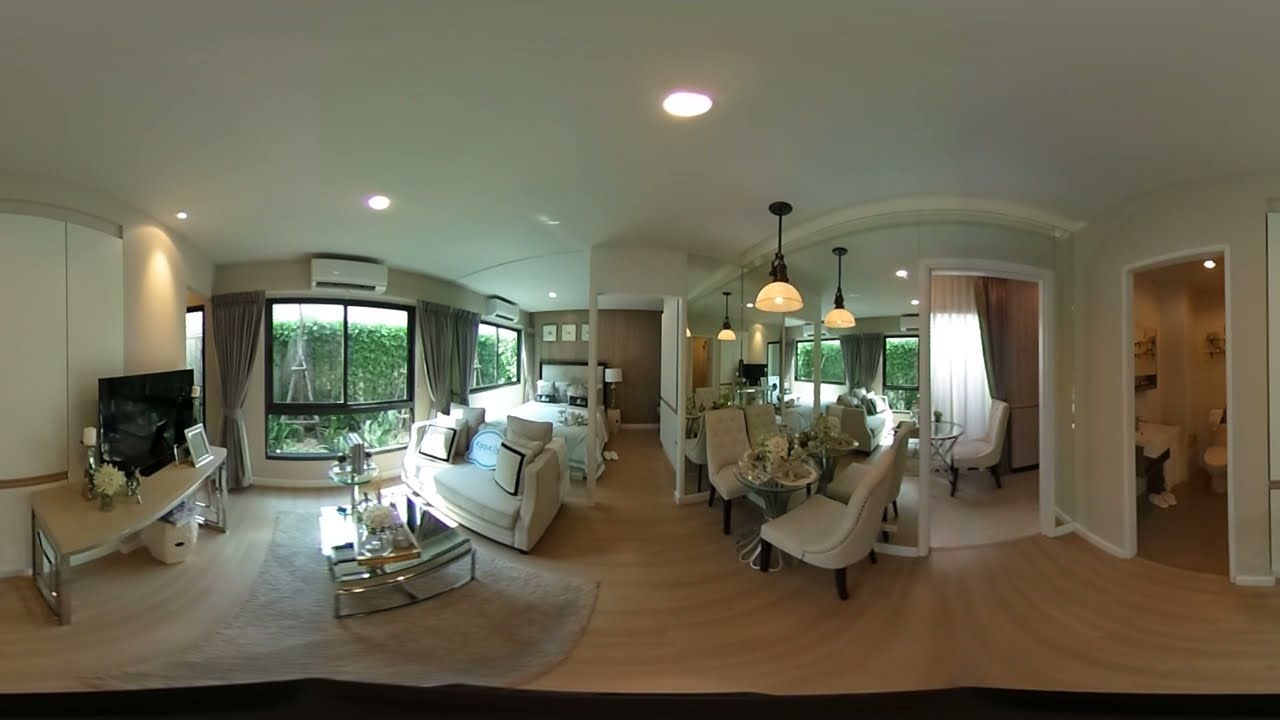The image showcases a spacious and well-lit living room, depicted during the daytime, with sunlight streaming in through large windows that dominate one side of the space. These windows, framed with black and bordered by dark gray curtains, offer a view of lush green shrubs outside.

The flooring is a light brown, paneled hardwood, complemented by a strategically placed rug. The walls and ceiling are painted white, with the ceiling adorned by circular recessed lights and a single, black and white hanging light fixture over one of the tables.

The room features multiple furniture pieces including several couches and a bed visible in the distance, suggesting that this might be a hotel suite. A light-colored coffee table made of glass, with flowers in a vase, serves as a central piece. Near the windows, a table with silver legs and a white tabletop supports a large black flat screen TV. In front of the TV is a silver-framed picture.

Additional decor includes various picture frames, flowers in a vase, and a mirror that reflects the room's elements and opens up the view into another room. There is also a chandelier positioned above a set of chairs and a dining room visible beyond the mirrored area. To the side, a small, open bathroom with a white toilet and sink can be seen. An air conditioning unit is mounted above the windows.

Overall, the room exudes an inviting and luxurious ambiance with its elegant furnishings and meticulous detailing.